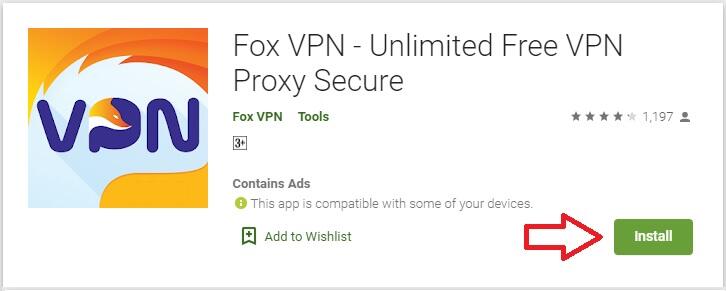This image features an app listing on a digital device interface. On the left side of the image is a square icon, which is visually segmented into sections. The top part of the icon is covered in wave-like patterns of orange, while an orange streak emerges from the bottom right, extending downwards about halfway. The color transitions to brown on the left side of the icon.

Beneath the icon, the app's name is displayed in blue letters. The letters include a "B," and possibly an "A," "P," or "N." Interestingly, a fox's face appears within the second letter, effectively splitting it. To the right of the app icon and name, the app is titled "Fox VPN - Unlimited Free VPN Proxy Secure," followed by a repeated mention of "Fox VPN." This section indicates that the app is categorized under "Tools."

The app has garnered four stars from 1,197 reviews and contains ads. A note at the bottom states that the ad is compatible with some of your devices. Below this information, there is a bookmark icon labelled "Wishlist." Further to the right of the bookmark icon, a large red-outlined arrow points towards a green "Install" button with white lettering.